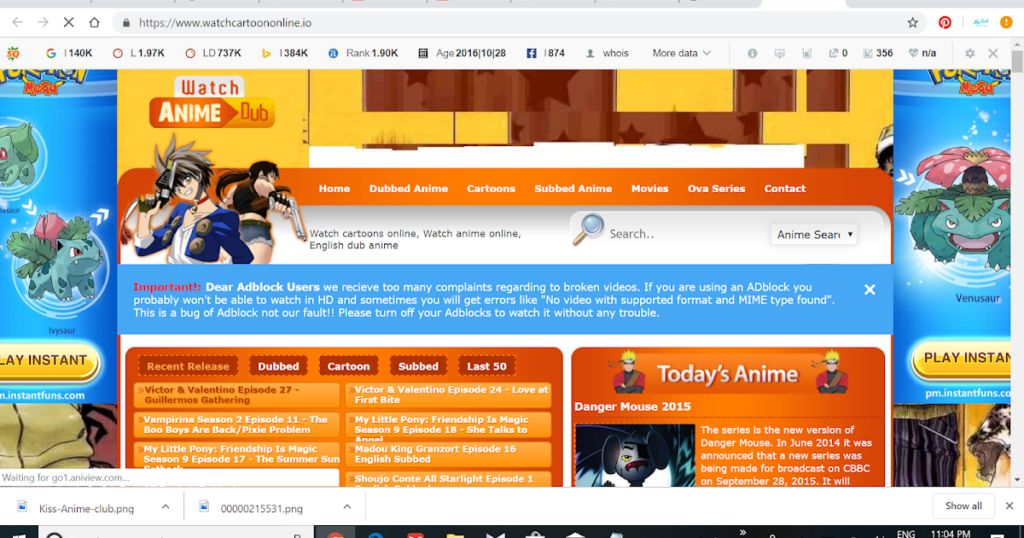Title: Detailed Summary of watchcartoononline.io Webpage Interface

Caption: The screenshot showcases the homepage of the website watchcartoononline.io. In the upper right corner of the page, several numerical values and abbreviations are displayed prominently:
- **SQ:** written in orange
- **G:** associated with 4DK
- **L:** marked as 1.97K
- **LD:** displayed as 737K
- **B:** represented with a yellow logo, labeled at 4K
- **A:** indicated with a blue "A" and recorded as 1.90K
Additionally, below the title, there appears to be metadata indicating a date of *October 28, 2016*, along with a Facebook reference tallying up to *874* likes. 

Central to the page is a bold and colorful heading, "Watchanimdab," printed in a striking combination of red, orange, and white text against a white background. Below this are navigational tabs for various sections of the site, including:
- **Home**
- **Dubbed Anime**
- **Cartoons**
- **Subbed Anime**
- **Movies**
- **Ongoing Series**
- **Contact**

These tabs are set on an orange strip with white text. Following the tabs, the website encourages users with phrases: "watchcartoonsonline," "watchanimonline," and "englishdubanim."

A search bar with an accompanying magnifying glass icon is centrally placed for ease of navigation. Below this is an important red banner message for Adblock users, stressing the impact of Adblock on the viewing experience:
**“Important: Dear Adblock users, we received too many complaints regarding broken videos. If you are using an Adblock, you probably won't be able to watch in HD and may encounter errors like 'no video supported format' and 'MIME type not found.' This is a bug of Adblock, not our fault. Please turn off Adblock to watch without any trouble.”**

At the page's bottom, various anime thumbnails are presented against an orange background, further inviting users to explore the content offered by the site.